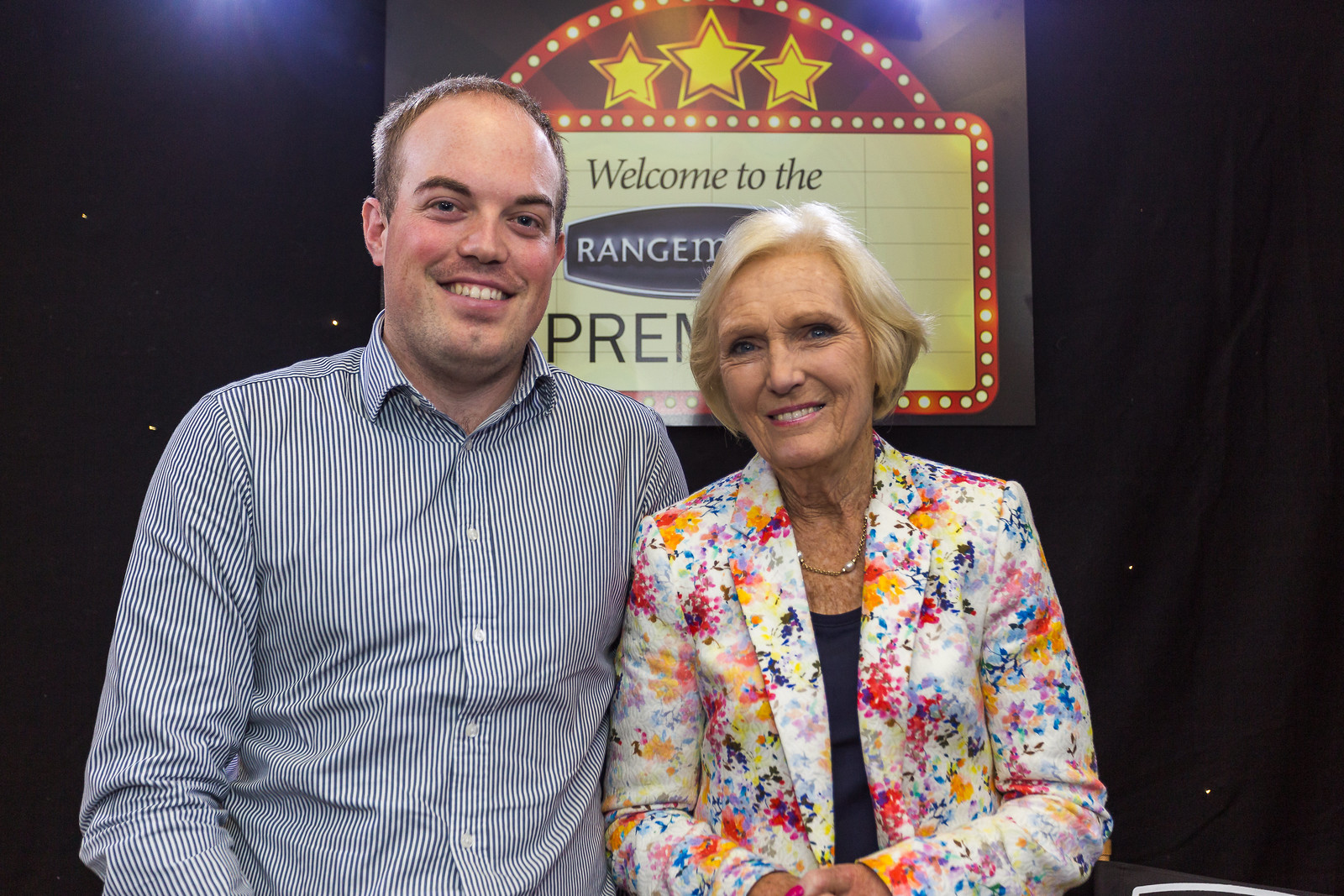In the image, two people are sitting next to each other against a dark background dotted with a few yellow specks of light. The person on the right is an elderly woman with short blonde hair, parted on the right and covering her ears. She has light pink lipstick on, showcasing her front teeth as she smiles warmly, her wrinkled skin, especially around her eyes, adding character to her expression. She is dressed in a white floral jacket over a dark shirt and wears a gold necklace draped over her chest. Her hands are clasped together on her lap. 

Next to her, on the left, is a younger man with a receding hairline wearing a long-sleeve blue and white striped button-up shirt. He also smiles broadly, showing his top row of teeth. He has brown eyes and eyebrows, and his gaze is directed toward the viewer. 

Behind them, a partially obstructed illuminated rectangular sign is visible, reading "Welcome to the" with the letters "R-E-N-G-E-M" and "P-R-E-M" partially covered by the woman's head. The sign features three yellow stars at the top, with the middle one being slightly larger, all encircled by an orange border with yellow dots and a rounded orange top with white dots. This color photograph is taken in landscape orientation, capturing the warm connection between the two subjects in a realistic and detailed style.